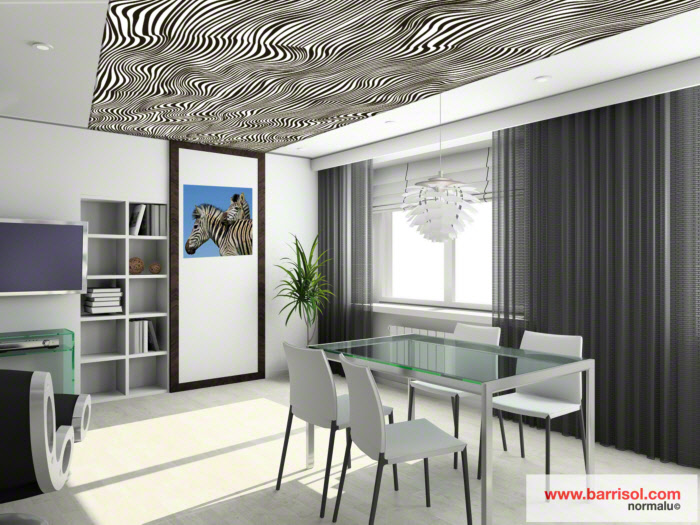The image showcases a stylish, contemporary living-dining room that could easily be featured on an interior design site. Dominating the foreground is a rectangular glass dining table surrounded by four white chairs, each with simple designs and four legs. To the right, an expansive window fitted with sleek black blinds allows natural light to flood the space, and above the dining table, a decorative art-deco lamp resembling an artistic rendition of a pine cone hangs elegantly. 

The ceiling features a unique zebra-striped pattern running through its center, with white or off-white sections flanking either side, accompanied by integrated lighting. On the left side of the room, a picture of zebras hangs on a white and black wall next to a well-stocked bookshelf with various items on its shelves. Nearby, a large green plant adds a touch of nature to the indoor setting. Centrally positioned on the back wall is a big screen TV set atop a glass table, which also holds a DVD player or DVR.

Additionally, parts of the room appear to be rendered, which could indicate a computer-generated design plan. Text in the bottom right corner reads "www.barrisol.com" in red, with "N-O-U-R-M-A-L-U ©" in black beneath it. In summary, the room features a harmonious blend of modern elegance and artistic accents, creating an inviting living-dining space.